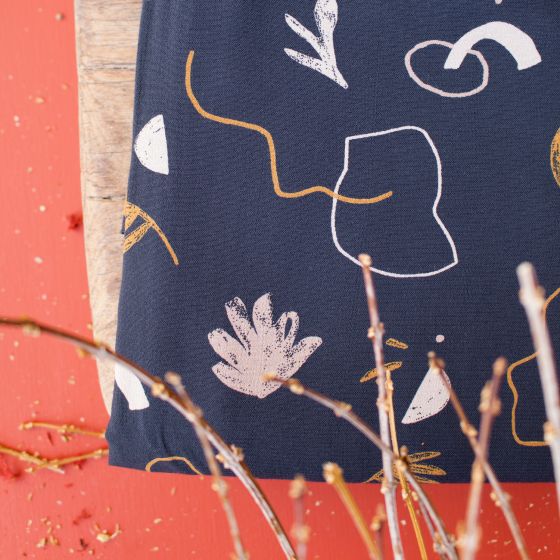This detailed color photograph features a blue, canvas-like fabric adorned with various patterns and designs, primarily in white and yellow. The designs include white leaf patterns, a white semicircle, a three-leaf motif, a white circle with a crescent emerging from its center, and a white line intersected by a yellow line. The fabric appears to cover the majority of the image and may be either folded to reveal a flat, wood-like underside or double-layered with such a base. Beneath this fabric lies a damp, orange-red surface scattered with plant debris, including small, light brown to almost white branches and twigs. These plant stems extend from the bottom right corner, protruding into the frame, adding intricate texture to the scene. The overall setting is enriched with fine details such as broken pieces and granules on the red background, enhancing the photograph's complex and layered composition.